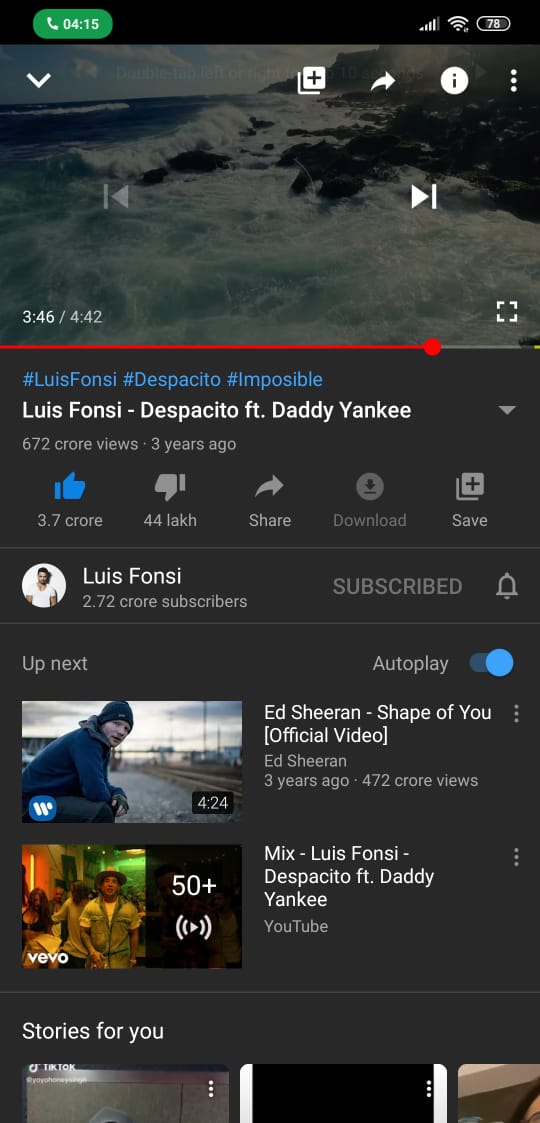This is a detailed screenshot from a mobile phone displaying a YouTube video within the app. The screenshot, taken while connected to a Wi-Fi network as indicated by the signal icon in the top-right corner, also shows the phone's battery at 78%. A green button with a phone icon and a timer in the top-left corner reveals that the user is on a call lasting 4 minutes and 15 seconds.

The paused video is of the music track "Despacito" by Luis Fonsi featuring Daddy Yankee, currently stopped at 3 minutes and 46 seconds. Uploaded three years ago, the video has accumulated 3.7K likes and 44 dislikes. Luis Fonsi's profile icon is visible, along with suggested "Up Next" videos, which include Ed Sheeran's "Shape of You" and a mixed Luis Fonsi playlist. The page also contains non-English text, indicating that the interface may be set to a different language.